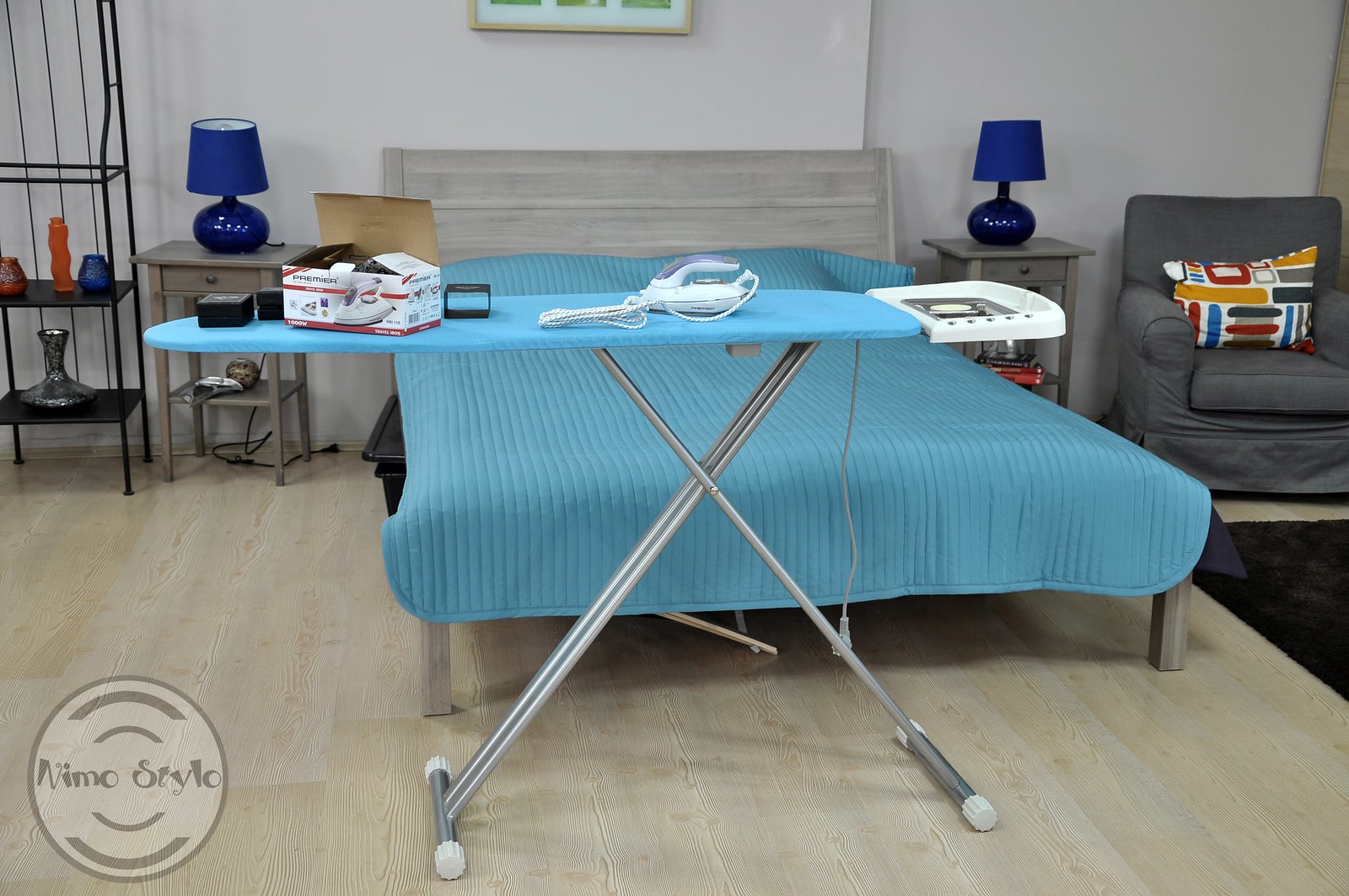The photograph captures a neatly arranged room dominated by a bed with an ash-gray headboard and a blue-green comforter. In front of the bed is a new ironing board, identifiable by its greenish-blue stretch cover and crisscross metal legs, equipped with floor-protective bumpers and a plastic stand for holding the iron upright. Atop the ironing board sits an unopened box for a very compact electric iron, which is also prominently featured. The room boasts two small gray end tables flanking the bed, each adorned with blue-shaded lamps, and a cushy dark gray armchair with a multicolored pillow near one of the tables. To the far left is an iron rod knickknack shelf displaying decorative blown glass items, including an orange vase and a short blue decoration. The synthetic wood grain floor is partially covered by a throw rug on the right side of the image, and in the bottom left corner, a circular logo with the text "NEMO Style" (or a variation of the name) is evident.